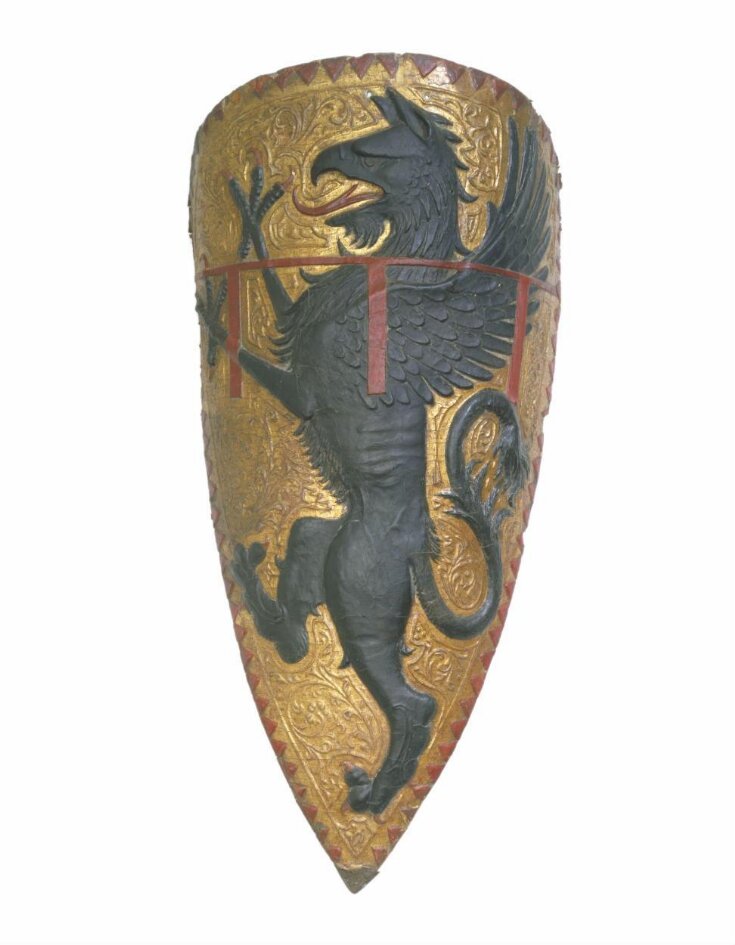This is a highly detailed color photograph of an ornate, ceremonial battle shield displayed against a white background. The shield has a distinctive shape, arrow-like with a pointy bottom and a strongly curved top, resembling a tall, narrow form. The overall surface is richly adorned in gold, featuring intricate and stylized botanical motifs of flowers and branches in elegant engravings. The center of the shield prominently displays a black griffin—a mythical creature with the head of a hawk, complete with pointy ears, and the body of a lion. The griffin's mouth is open, revealing a red, snake-like tongue. Its wings extend to the right. Adding to its grandeur, there are red triangular accents around the edge of the shield, culminating in a gold tip at the bottom. The griffin's tail, which curls towards the right, is also detailed with spikes, contributing to the overall intricacy and mythological essence of the shield's design.